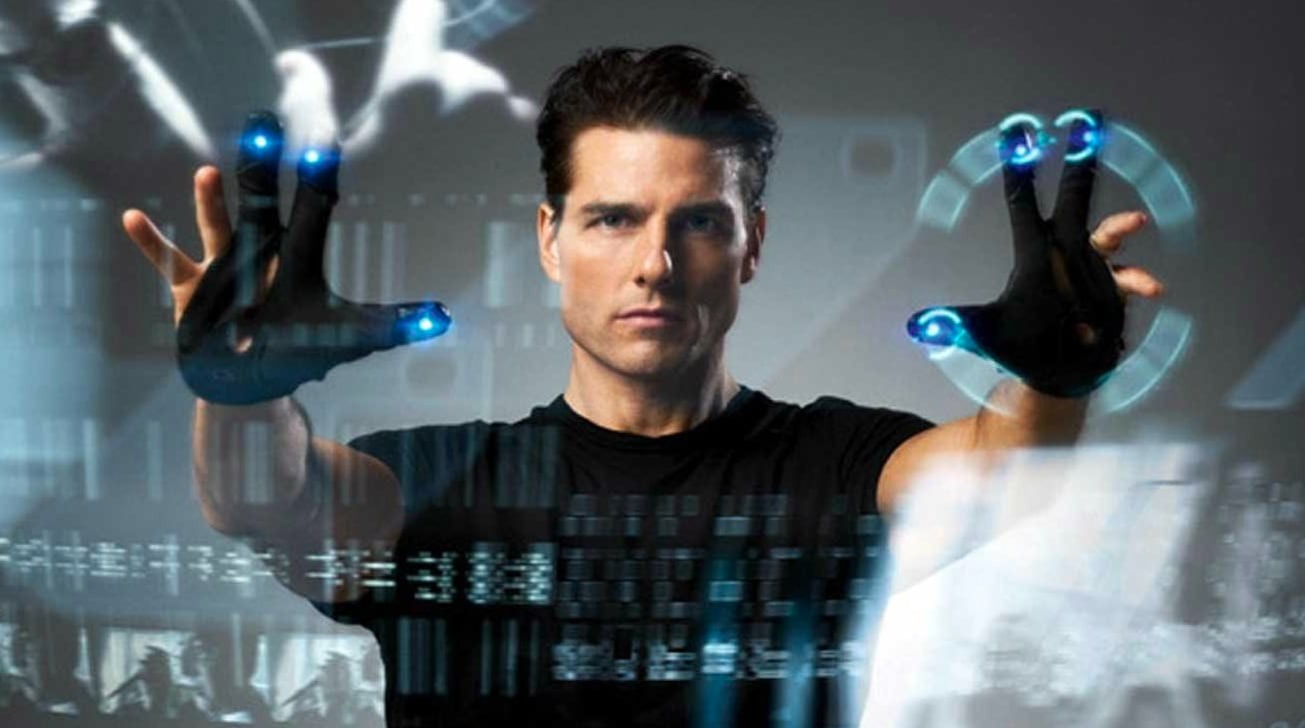This photograph is a still frame from the movie "Minority Report," featuring Tom Cruise. The image centers on Cruise, who is a white man with a fairly tan complexion and dark brown hair. He is clean-shaven and sports a muscular jawline. Cruise is wearing a black short-sleeved shirt and high-tech gloves on his hands. The gloves are predominantly black and feature blue lights at the fingertips. These gloves only cover his middle, pointer, and thumb fingers, leaving his pinky and ring fingers exposed.

In the frame, Cruise is facing the camera with his hands outstretched in front of him, appearing to interact with a futuristic, transparent interface. He is seemingly trying to decode or manipulate something on the pane of reflective glass using his gloves. At the bottom part of the photograph, a turquoise pixelated light adds a digital ambiance to the scene, emphasizing the advanced technology he is engaged with. The strong visual cues and Cruise’s intense expression suggest he is in a moment of critical operation within the sci-fi narrative of the film.